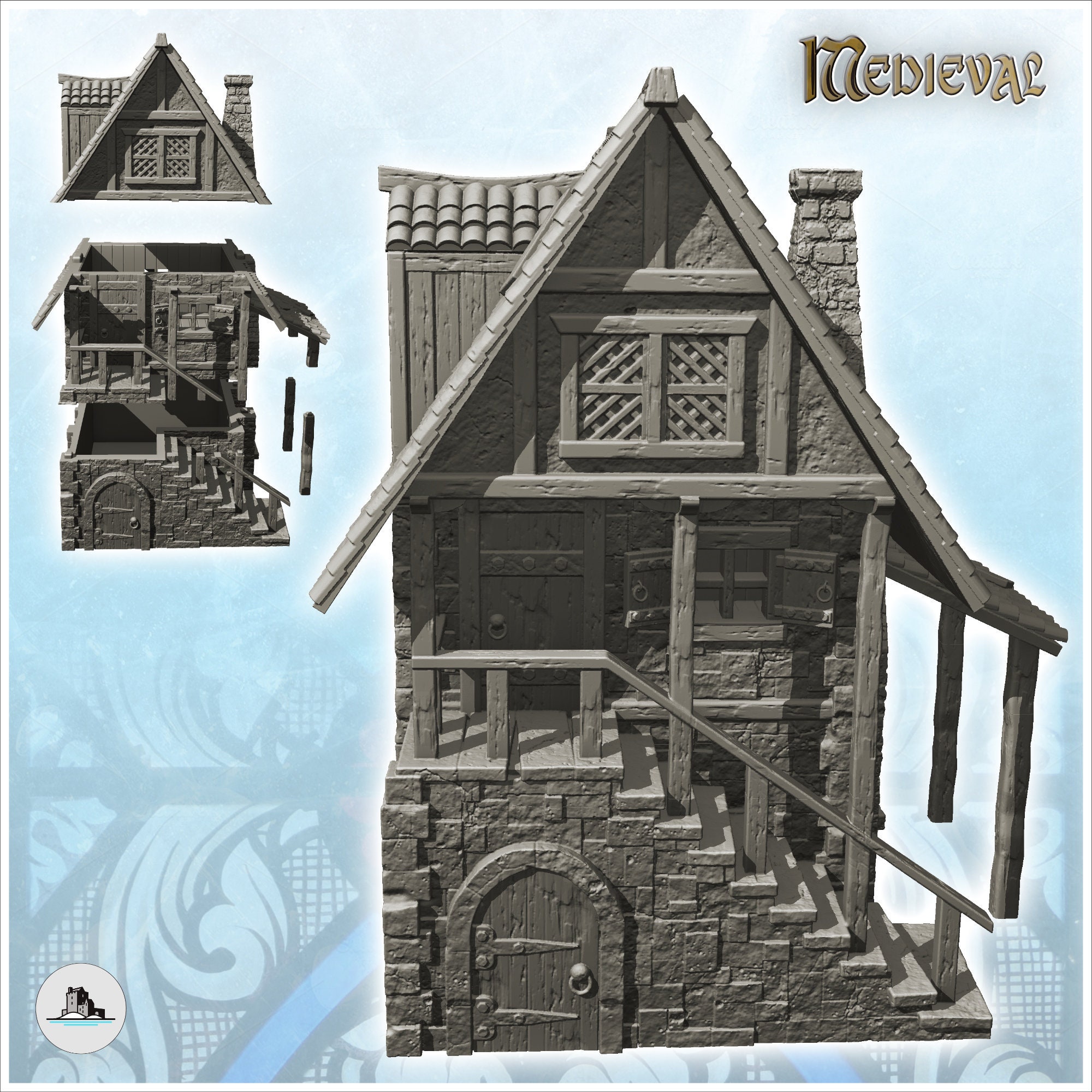The image showcases a detailed 3D model of a two-story medieval house, rendered in grey. The model, resembling an assembly kit, features intricate craftsmanship, particularly notable in the arched door on the ground floor. The house includes a set of stairs leading to an upper-level entrance, and the roof is triangular with tile detailing. The model's left side reveals a segmented view of the floors, emphasizing its layered structure. A large double window is prominent on the second floor, adding to the architectural authenticity. The background is bluish, with the word "medieval" in brown, prominently displayed in the upper right corner, enhancing the historical context of the model.